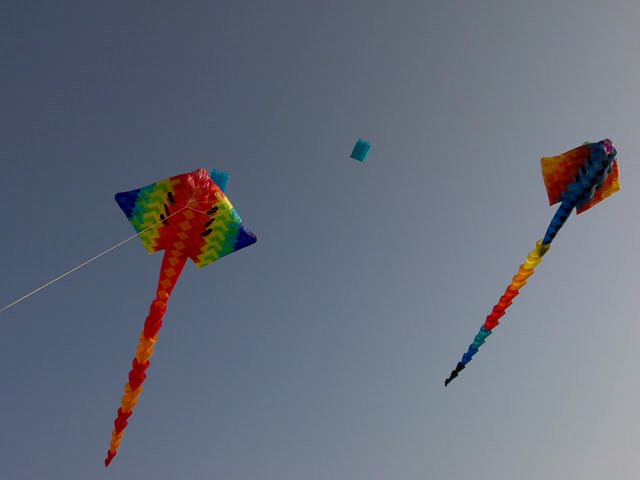The photograph captures a clear bluish-gray sky with two vibrant, pillowy kites soaring high. The kite on the left showcases a rich rainbow of colors: its center is an orange hue adorned with yellow rhombuses; the wings display a striking array of yellow, green, sky blue, and dark blue, and at the top sits a turquoise rectangle. Its tail, elegantly flowing, alternates between shades of red and marigold yellow. In contrast, the kite on the right features a dark blue center with black rhombuses. Its wings are a brilliant mix of red, yellow, and orange, complemented by a tail of dark blue, yellow, orange, red, turquoise, and black. A distinctive turquoise rectangle is also seen floating nearby. The white string of the left kite is clearly visible, trailing it as it dances through a sky that varies from medium dark blue to sunny gray, indicating either midday or twilight.